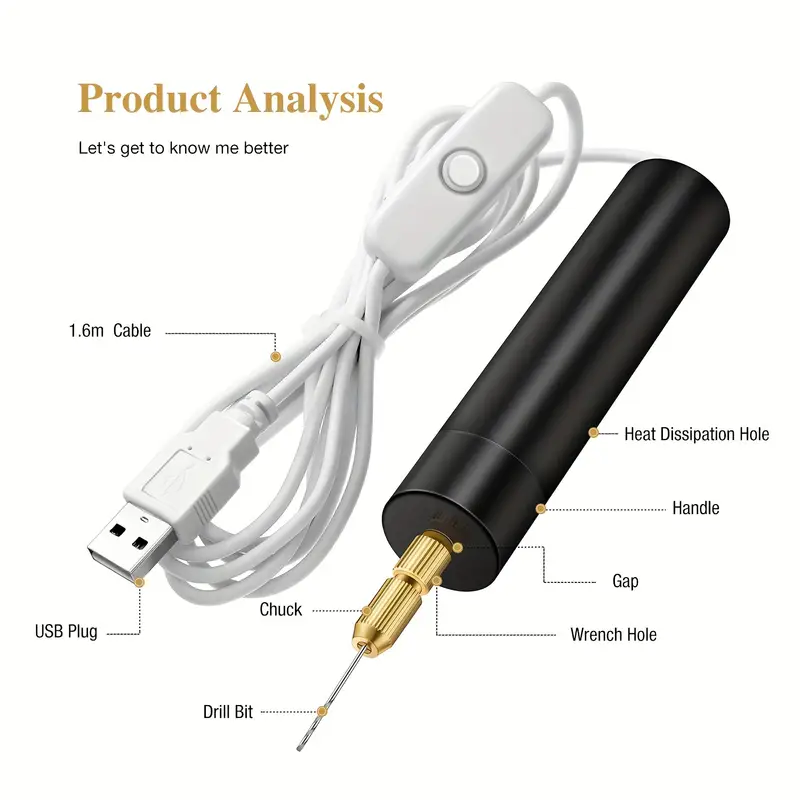The image is set against a white background, showcasing a small electronic tool with a white USB cable attached. At the top left, "Product Analysis" is printed in gold, followed by the smaller black text, "Let's get to know me better." The product features a black, wide cylindrical base connected to a white, 1.6-meter USB cable with a small button on it. The tool on the right, which appears to be a USB-powered drill, has a silver drill bit and a gold-plated chuck. Various areas of the device are labeled in black text, including the drill bit, chuck, wrench hole, gap, handle, heat dissipation hole, USB plug, and the 1.6m cable, helping to identify the components and functionality of the tool.